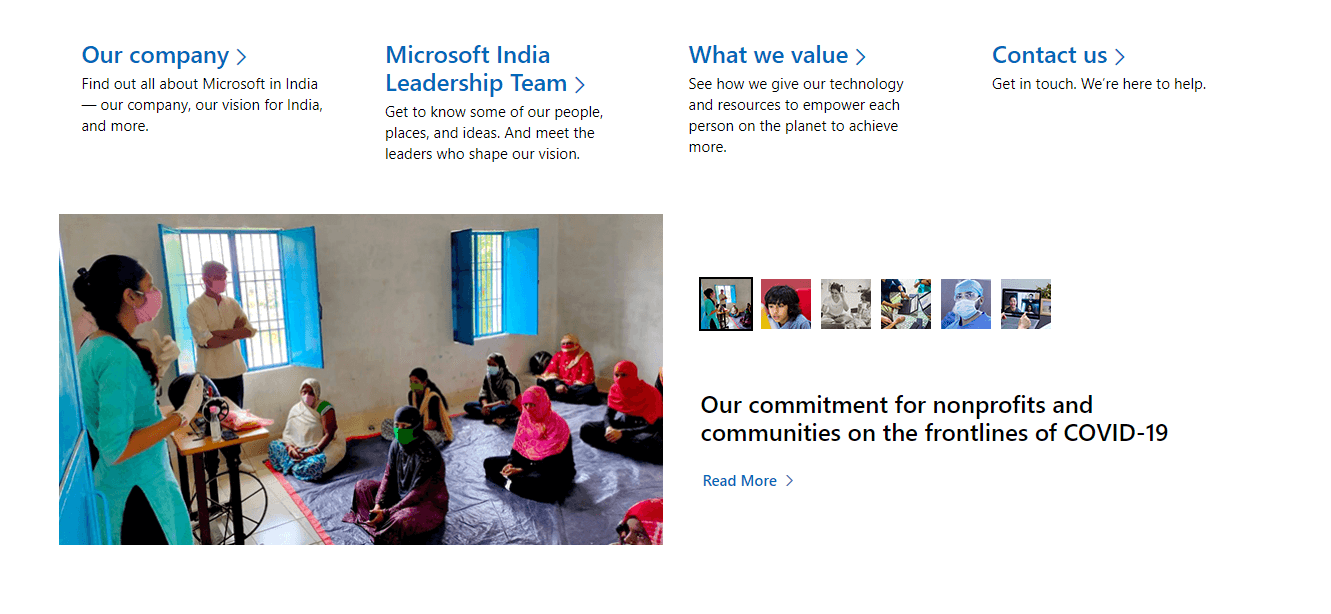**Caption:**

On a dedicated webpage featuring a clear, white background with blue lettering, the mission and efforts of Microsoft India are prominently highlighted. The main headline invites visitors to "Find out all about Microsoft in India," covering detailed sections about the company's vision and its leadership team in India. 

One of the focal points is a heartwarming large image where a woman dressed in a blue dress, with a ponytail, and wearing a pink face mask and white gloves, is seen engaging with a group of young female students. These students, all seated on a floor mat, are wearing different variations of the hijab. This specific scene reflects Microsoft's commitment to inclusive education and community support.

Supplementary smaller images illustrate Microsoft's support for nonprofits and communities, especially those on the front lines of combating COVID-19, with a call to action labeled "Read more."

The webpage emphasizes the company's values, showcasing how Microsoft deploys its technology and resources to empower individuals globally. Additionally, there is a "Contact Us" section, encouraging visitors to reach out for assistance.

Overall, it serves as an advertisement illustrating Microsoft's initiatives and contributions within India.